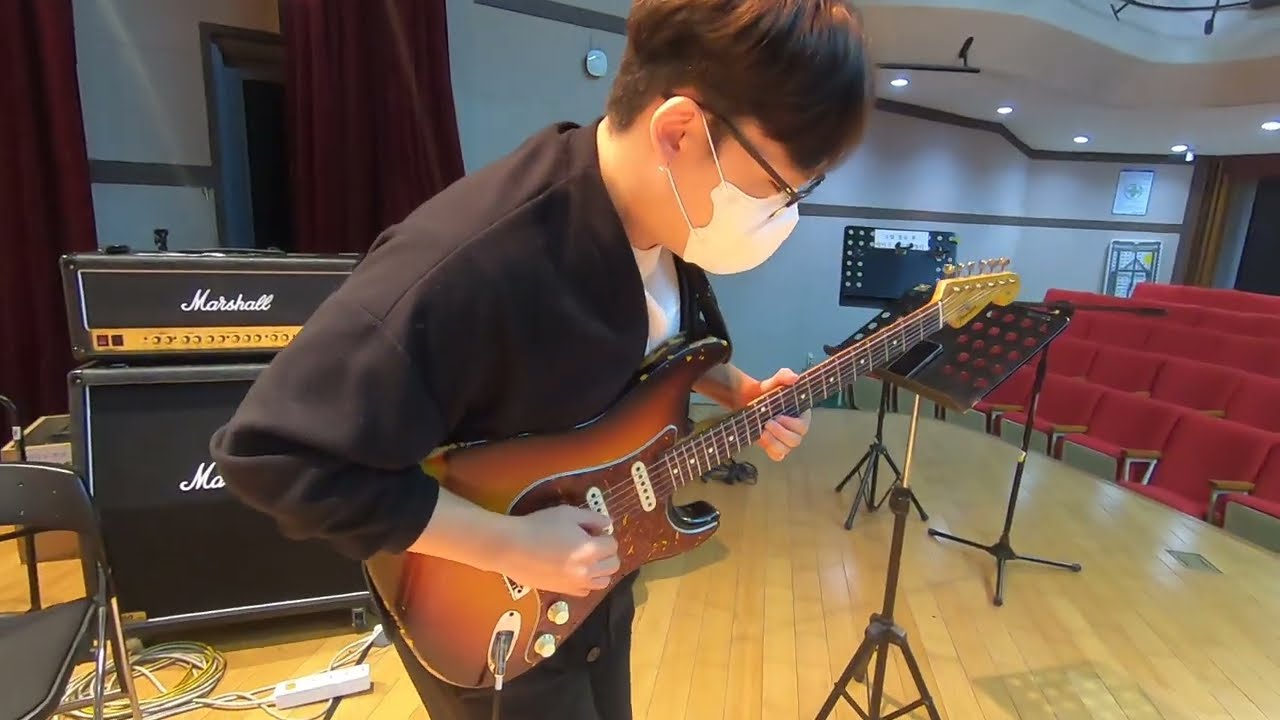This color photograph, captured in a landscape orientation, depicts an indoor auditorium scene with a focus on a young male guitarist, approximately 16 years old, standing center stage. He has short dark brown hair, wears black glasses, and a white facial mask reminiscent of a hospital mask. The young man is dressed in a black jacket over a white t-shirt and black pants. He holds a brown electric guitar, strumming it with his right hand while his left hand manipulates the fretboard, the neck of the guitar pointing toward the right side of the image.

The stage itself is constructed from honey-colored oak planks, giving it a golden hue. On the right side of the guitarist, there are several black music stands and microphone stands. To his left, a Marshall amplifier stack rests nearby, accompanied by a black leather-covered chair. The floor in front of this setup is scattered with white cables. 

In the distance, there are about four or five rows of red auditorium seats, partially visible on the right side of the image. Red theater curtains hang on the left side of the stage, contrasting with the white walls that feature a horizontal gray stripe. Overhead, ceiling lights illuminate the scene, enhancing the realistic representation and detail of this photorealistic image. Scattered signs decorate the walls, adding to the ambiance of this small yet detailed venue.